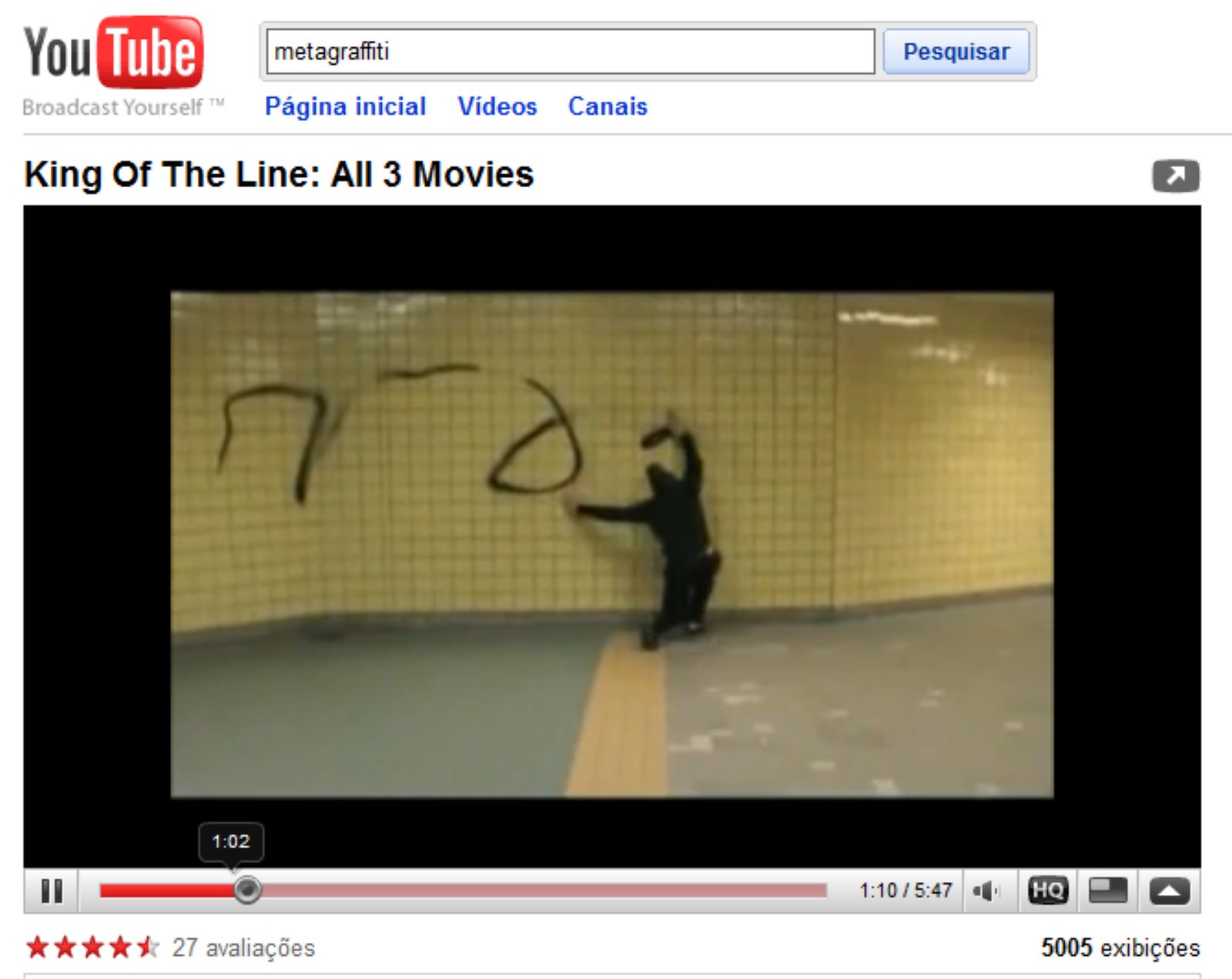This is a detailed screenshot of a paused YouTube video titled "King of the Line: All Three Movies," stopped at the 1:02 mark. The YouTube interface is visible, with the distinctive YouTube logo in the upper left corner. Next to the logo, the search bar contains the term "Meta Graffiti" and the button labeled "Pesquisar," indicating the language setting is not English. Below the search bar are navigation options labeled "Página Inicial," "Vídeos," "Canais," and "Canet." 

The video itself shows a man dressed in black, including a hoodie, sweatshirt, pants, and tennis shoes, spray-painting black scribbles on a wall made of shiny yellow tiles, suggesting that this is in a subway station. The graffiti appears random and non-artistic, and the scene feels more like vandalism than creative expression. The video is rated four and a half stars out of five, with 27 likes visible, and standard YouTube buttons such as quality settings (HQ) can be seen on the screen.